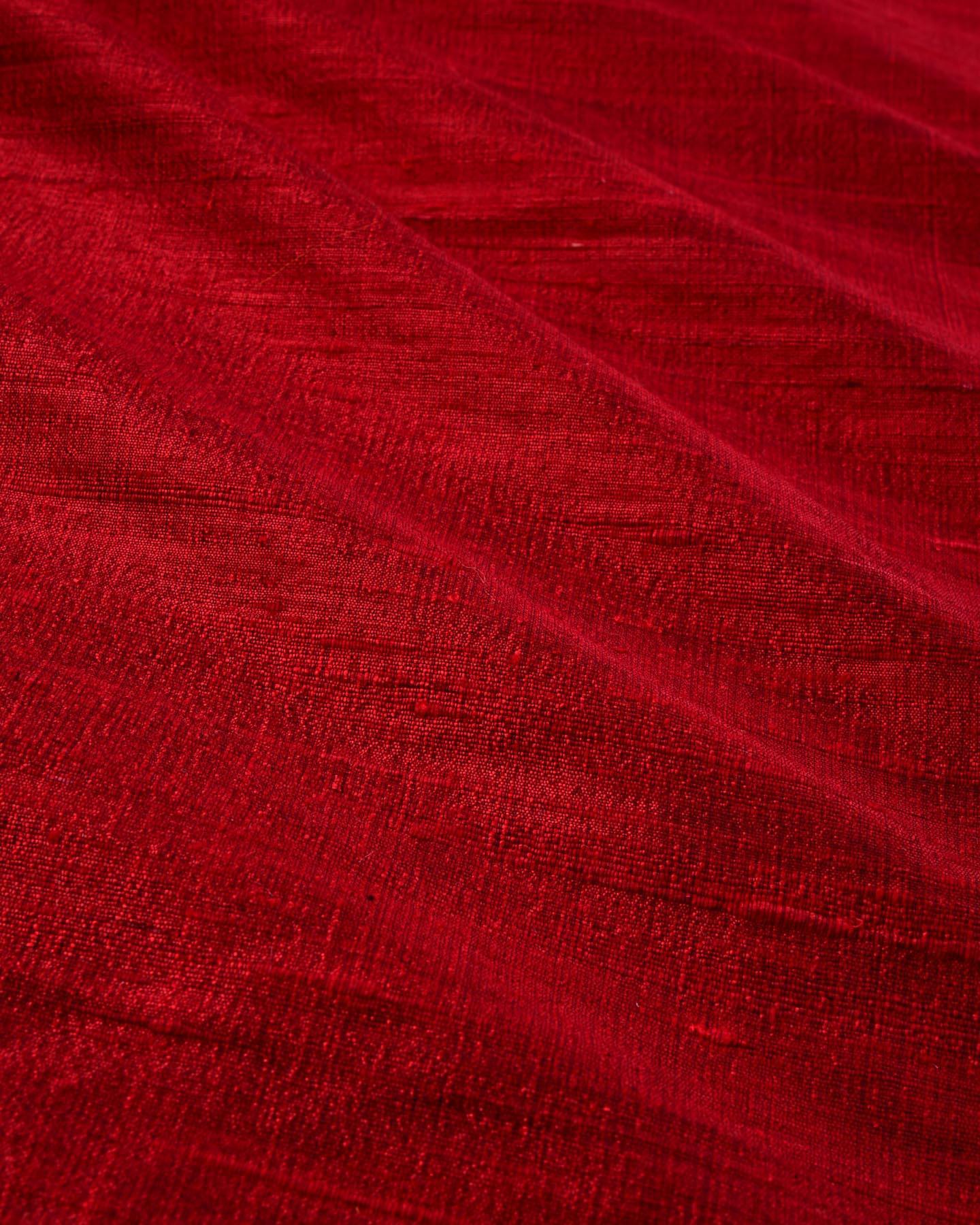The image depicts a rich, maroon red fabric, possibly resembling burlap or linen due to its evident texture. The fabric is laid out in a rectangular shape, with its shorter sides positioned horizontally at the top and bottom. The top left and bottom left areas of the fabric are slightly darker, influenced by the lighting and angles of the camera capturing the scene. 

From the top right corner, there are six distinct folds that create undulating waves across the fabric. The first two folds extend diagonally from top to bottom, spanning the entire width of the fabric. The third fold emerges primarily in the bottom right quadrant, fading out towards the top left center. The fourth fold, the thickest one, begins at the top left corner, splits midway, and reappears slightly to the right, continuing down to the center. The fifth fold is visible only in its lower half, while the last fold stretches from the bottom right corner to about the midpoint vertically. 

The varying lighting reveals subtle shadows throughout the creases and folds, alternating between darker and lighter shades of red. This play of light and shadow accentuates the waves, making the texture more pronounced and giving the fabric a dynamic, three-dimensional appearance.